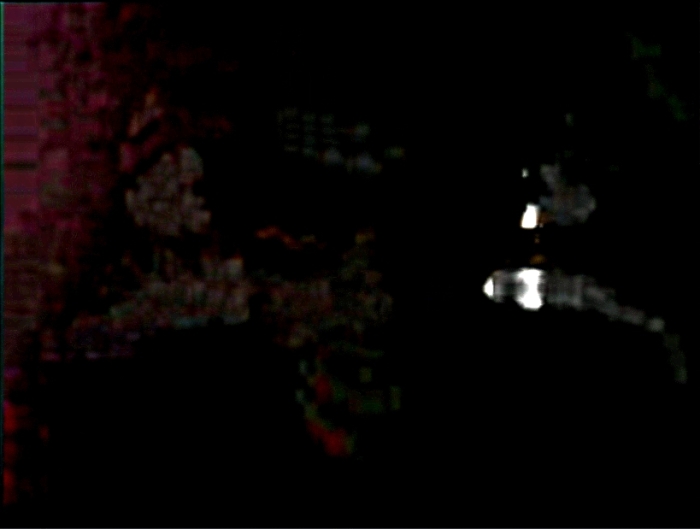In the image, we observe a predominantly dark scene that is somewhat ambiguous. The darkness is almost all-encompassing, evoking the impression of a photograph taken in a dim or obscured setting, possibly even as if captured accidentally. The left side of the image features an area where the darkness lightens and transitions into a red, glitching texture that stands out amidst the nearly impenetrable blackness. This red section appears blocky, with irregular shapes that suggest some kind of distortion.

To the right of this red glitch, there is a grayish texture that resembles a rock formation or a similar solid structure. Further to the right, the image hints at the silhouette of a person, possibly a woman. This figure is faint and grayish, standing out just barely against the darkness. Adjacent to this figure, there are small patches of white light, which could be from a flashlight or another source of illumination. These lights also appear to form shapes beneath the figure, enhancing the eerie quality of the scene.

Overall, the image is extremely dark, with scarce details that make identification challenging. The combination of red glitching textures, gray rock-like features, the faint silhouette of a person, and sporadic white lights suggest a scene that is both mysterious and unsettling.